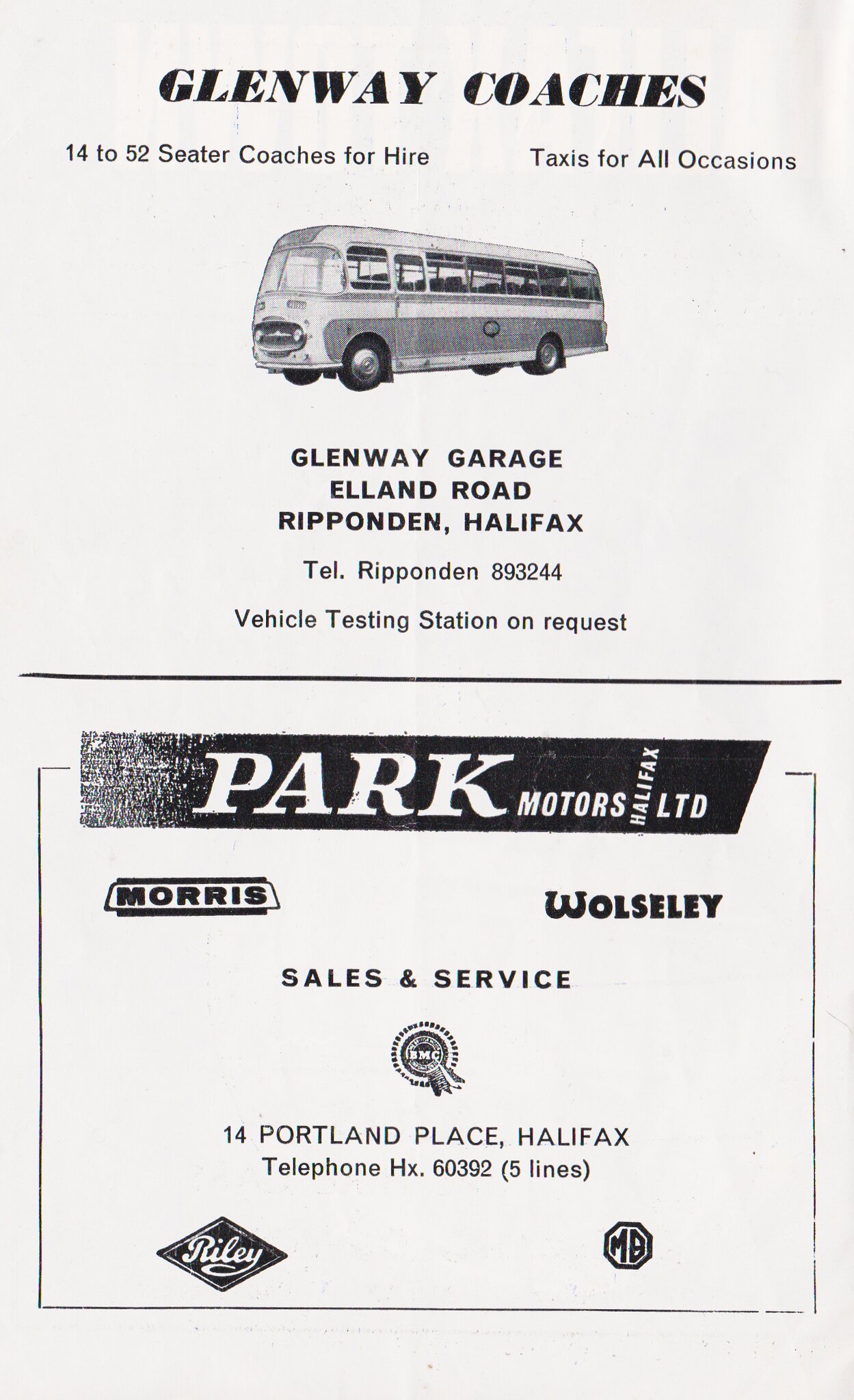The black-and-white advertisement appears to be a vintage flyer or brochure, featuring a nostalgic design reminiscent of the 1950s. The top section prominently displays the heading "Glenway Coaches." Below this, it states, "14 to 52 seater coaches for hire, taxis for all occasions." Accompanied by an image of a classic bus, the text further provides the company's address: "Glenway Garage, Elland Road, Ropondon, Halifax," and includes the contact number "Telephone Ropondon 893244." It also mentions "Vehicle testing station on request."

Beneath this advertisement, another section highlights "Park Motors Halifax Limited." It lists "Morris" on the left and "Wolseley" on the right, with the tagline "Sales and service" next to "14 Portland Place, Halifax." The contact telephone is given as "HX 60392." Two automotive icons, "Riley" and "MB," appear at the bottom, encapsulating the overall nostalgic black-and-white theme of the advertisement. The printed material combines elements from business cards and classic promotional brochures.